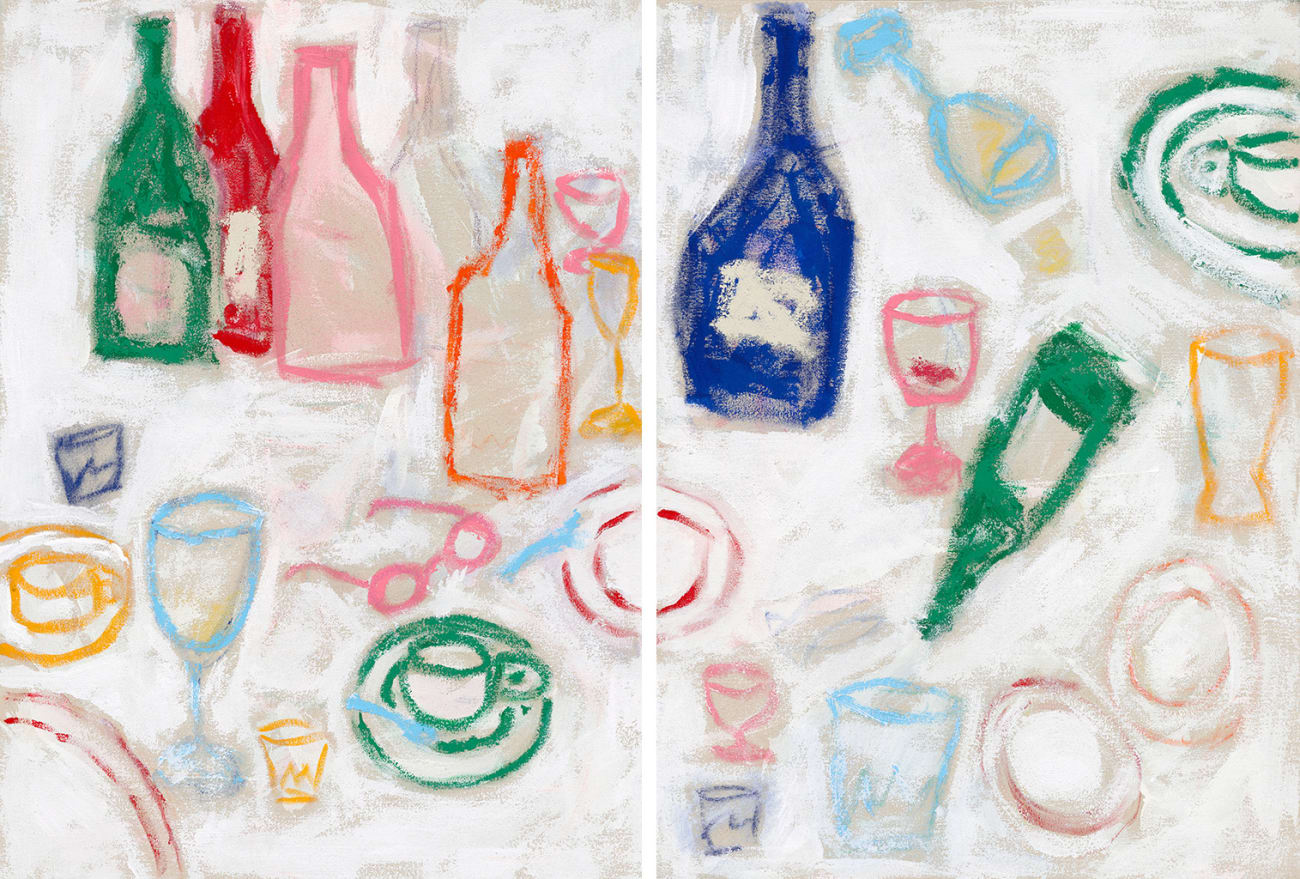The image showcases a detailed painting consisting of two complementary parts. Both parts sit against a white background with subtle tan hues. They depict an eclectic arrangement of various bottles, glasses, and dishware. On the left side, the background features:

- A green bottle with tan details
- A red bottle with white accents
- A pink bottle

Nearby, there is an orange-outlined bottle and a tan-outlined bottle. Following these, we see two drinking glasses: one pink and one yellow. A noticeable pink pair of eyeglasses is placed next to a green teacup set on a blue saucer, and another teacup set, which is yellow. A distinctive red plate is split between the left and right sections. 

Moving to the right image, the upper left showcases a blue bottle alongside a blue drinking glass lying on its side. Below it, a pink drinking glass sits next to a horizontal green bottle. The upper right corner contains another green tea set. The bottom right corner features two red dishes while the bottom left shows a pink glass beside two drinking cups: one dark blue, the other light blue. 

The painting, reminiscent of a whimsical, almost childlike, crayon drawing, blends impressionistic and abstract elements with its depiction of transparent and solid-colored objects outlined in orange, blue, yellow, and pink.